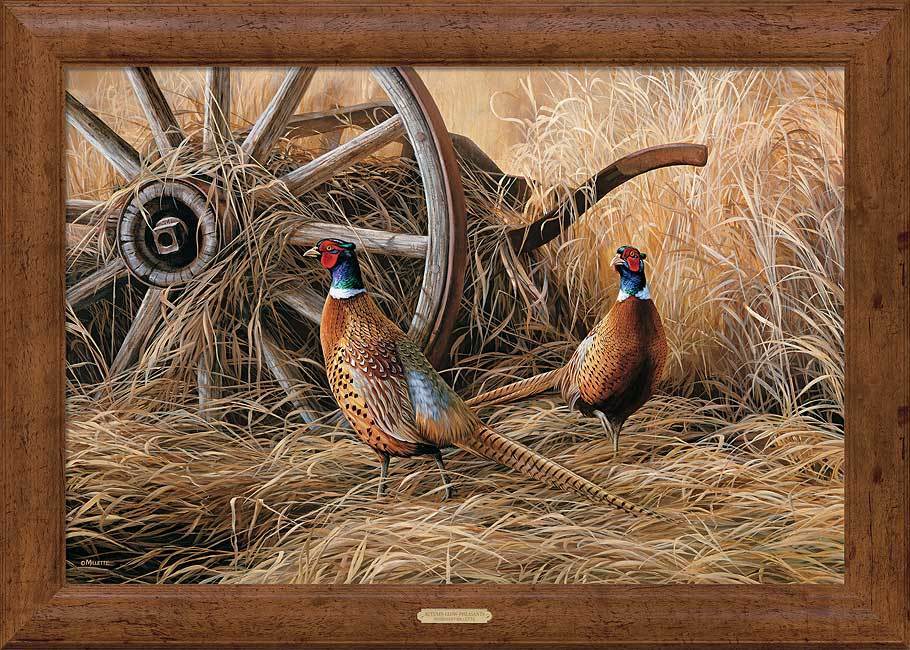The detailed oil painting is encased in a dark brown wooden frame, distinguished by an interesting grain pattern and an attached small brass nameplate whose inscription is unreadable. The artwork captures two ring-necked pheasants in a wheat field. The pheasants, centrally positioned, display striking features: brown bodies with polka-dotted chests, long striped tails, dark blue heads, and vivid red facial patches. One bird stands in profile, showcasing its sharp beige beak, while the other faces partially forward with one foot raised. The surrounding field is a blend of light tan hay and standing dried wheat, some of which appears trampled where the pheasants roam. In the background, there is an old wooden-wheeled farm implement, likely a thresher, characterized by unpainted wood and a steel-rimmed wheel. The painting's backdrop includes clusters of beige and white weeds, harmonizing with the overall golden tones, suggestive of a late summer harvest setting.